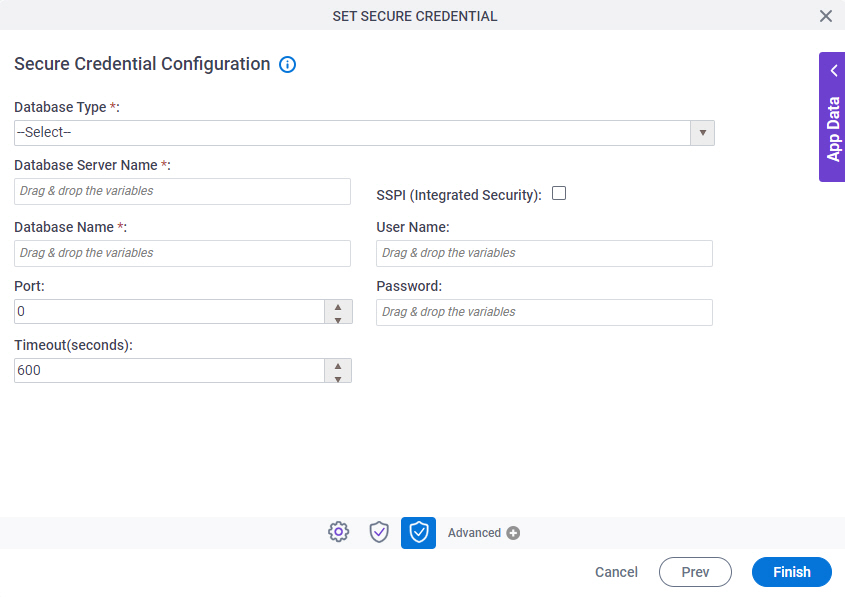This screenshot demonstrates a secure credential configuration interface with multiple drop-down menus and fields. The first drop-down menu allows the user to select the type of database. Directly below it, there is another drop-down menu for specifying the database server name, followed by a field for the database name. Users are instructed to drag and drop variables into these fields.

Subsequently, there is a prompt to select the port, which is currently set to 0. Below that, users can configure the timeout in seconds, with the default value set to 600. An option is available to enable SSP integrated security via a check box. If enabled, users can enter the username and password in the respective fields, again with prompts for dragging and dropping variables.

In the lower section of the interface, a light blue strip contains three icons: a gear, a shield with a tick, and another shield with a tick inside a blue square. At the very bottom right corner, there are three buttons for navigation and actions: a 'Cancel' button, a 'Previous Page' button, and a 'Finish' button.